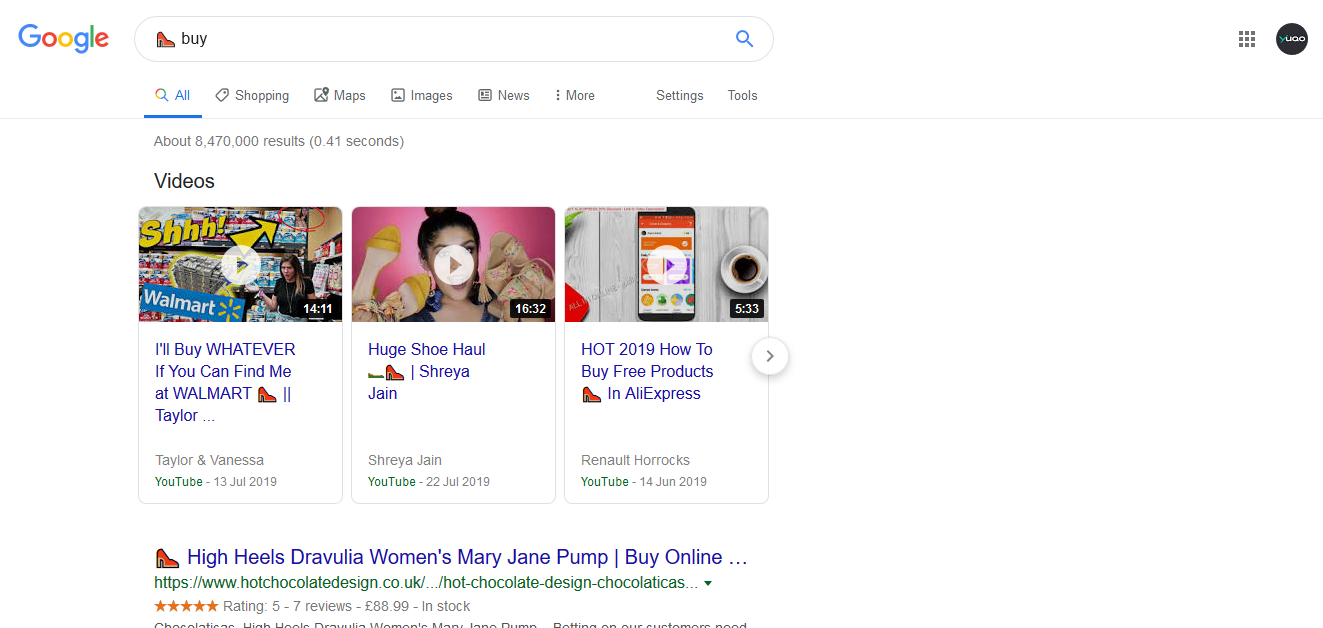The image depicts a Google search results page with a predominantly white background. At the top left corner, the colorful Google logo, featuring the letters "G," "o," "o," "g," "l," and "e" in blue, red, yellow, blue, green, and red respectively, is clearly visible. Adjacent to the logo is the search bar, which currently displays the query "buy."

Directly below the search bar are various navigation options including "All," "Shopping," "Images," "Videos," "News," "More," along with "Settings" and "Tools" menus. The active tab is set to "All," indicating that it encompasses all types of available results.

The search has yielded approximately 8,470,000 results in just 0.41 seconds. Prominently positioned near the top are three video thumbnails. The first video, titled "I'll Buy Whatever If You Can Find Me at Walmart," is followed by "Huge Shoe Haul,” and lastly, "Hot 2019 How to Buy Free Products on Aliexpress."

Below the video thumbnails, a search result for a product is displayed. It features high heels named "Druvillia Women's Mary Jane Pump." These shoes are available for purchase online at the URL: https://www.hotchocolatedesign.co.uk.